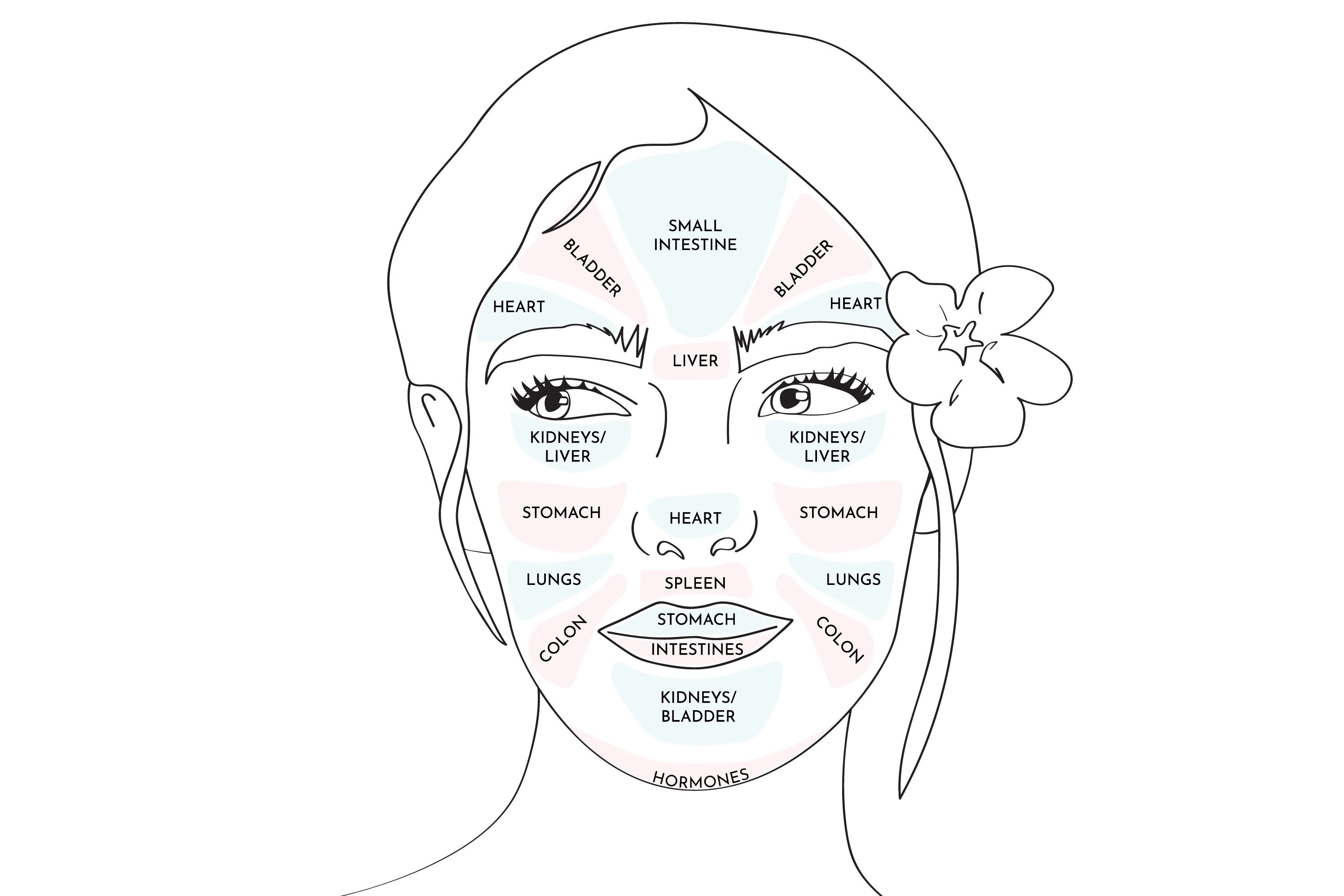This is a meticulously detailed black-and-white drawing of a woman's face, capturing her with a contemplative side-eye gaze directed to the left. Her hair is styled in a bun with a few loose strands, and a rose is elegantly tucked behind her left ear. The entire face is annotated with various body parts and organs, labeled starting from her chin and spiraling around. Starting at her central chin, the labels read hormones, followed upwards by kidneys and bladder. On her lower lip is the word intestines, and on her upper lip, the word stomach. Below her nose is labeled spleen, and on the center of her nose is heart, with liver written between the top of her eyebrows.

Moving outward, her right cheek displays the word stomach, with lungs written on both lower cheeks and colon below the lungs. Below her right eye, the words kidneys and liver appear again. Her forehead is labeled small intestine, flanked by bladder on each side. Above her left eyebrow is the word heart, and the same is repeated above her right eyebrow. Thus, text continues to label each section of her face, creating a comprehensive map of internal organs correlating to different facial regions. The drawing has subtle additions of light pink color amidst the primarily black lines, enhancing its delicate and thoughtful appearance.